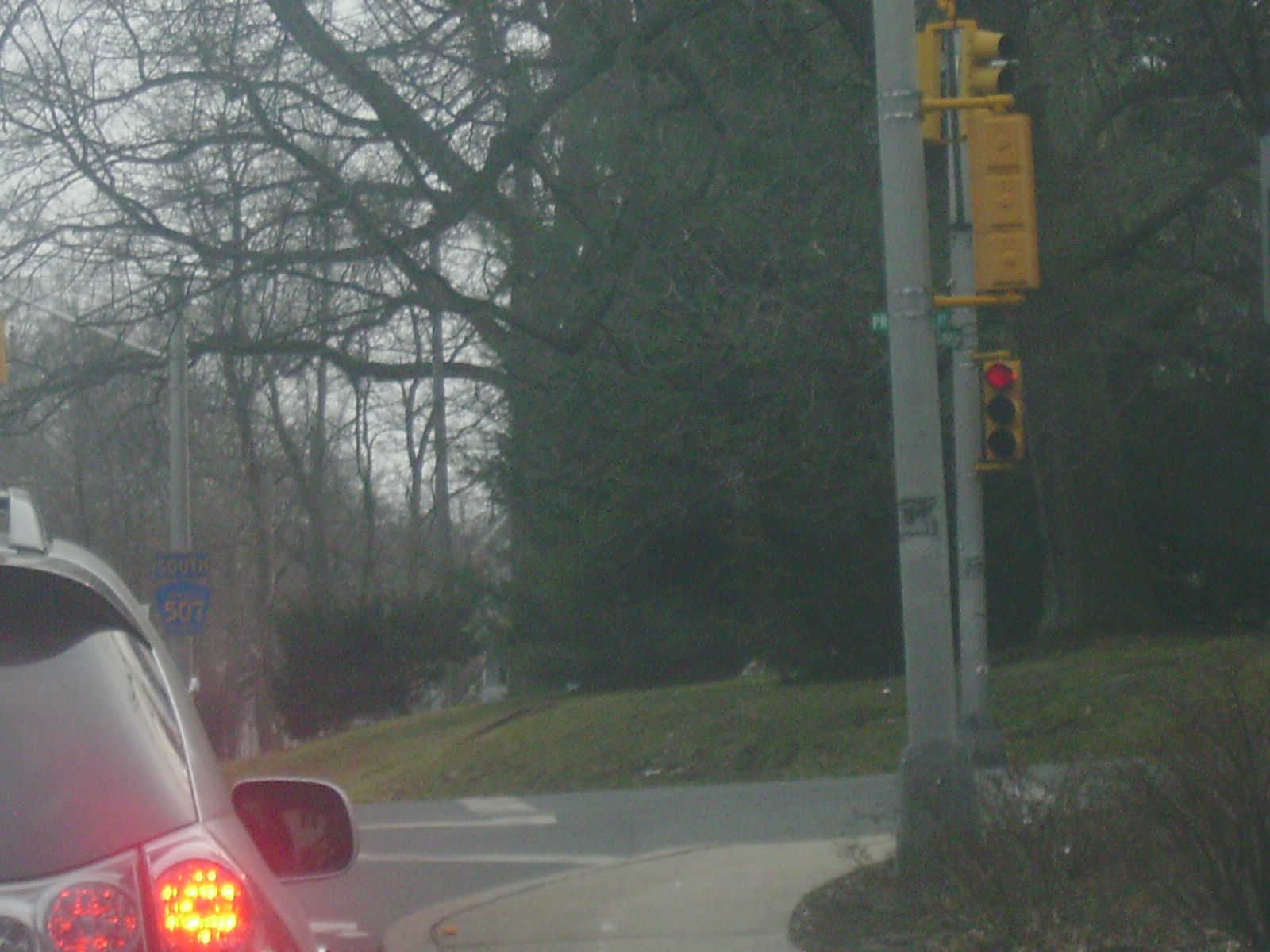This color photograph captures the rear corner of a vehicle in the bottom left-hand quadrant of the frame. A taillight emits a yellow glow while another, red taillight remains unlit beside it. The vehicle's rearview mirror is also visible. The background is dark and slightly blurry, shrouded in fog, lending an eerie, mysterious atmosphere to the image.

In the upper left of the frame, dense trees rise into the foggy sky, with patches of gray visible between their branches. Behind the thick tree line, a building is faintly discernible toward the right side of the image. Green grass carpets the ground beneath the trees, adding a natural contrast to the scene.

A road runs along the bottom of the photograph, marked by white lines, while a curved pavement borders the right-hand side. This pavement is adorned with some shrubbery, enhancing the natural elements in the frame. A large metal pole emerges from the right-hand pavement, topped with a rectangular yellow box. This box appears to support two traffic lights. The traffic light in view shows a red signal illuminated at the top, commanding attention amidst the foggy backdrop.